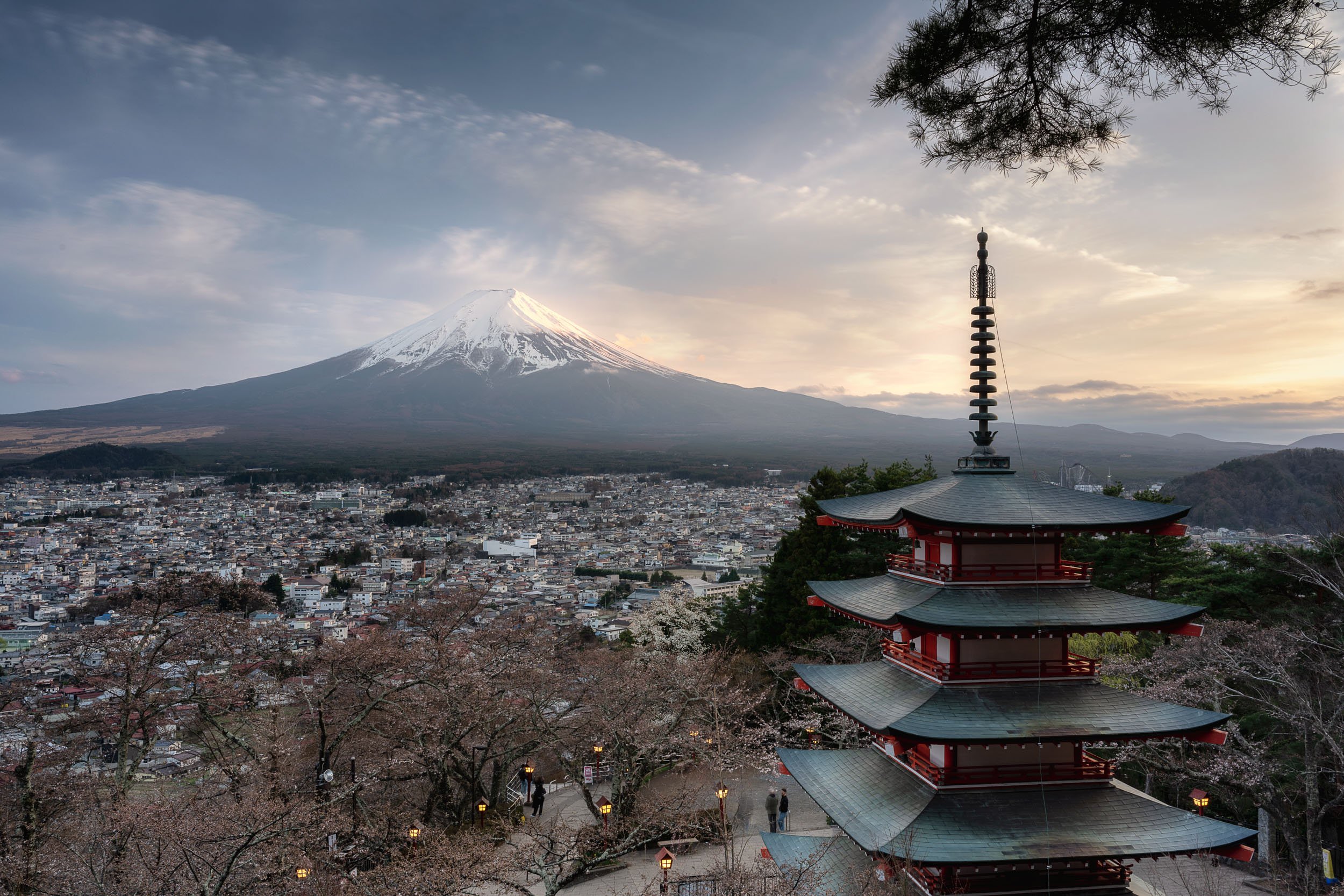This is an aerial photograph looking down on a bustling Asian cityscape, likely in Japan or China. Dominating the foreground is a striking, multi-tiered building with four visible stories and roofs extending outward in an umbrella-like fashion at each level. The structure is accented in red between the tiers and features a distinctive spiral or weathervane at its pinnacle. Surrounding the building are a few brushy, low-lying trees and various low lights, hinting at dusk with a subtly brighter sky on the right.

Stretching into the valley below, an immense expanse of hundreds, if not thousands, of densely packed buildings forms a congested urban landscape. The city appears intact but is tightly compacted, covering nearly the entire visible valley floor. Towering beyond the cityscape, a majestic mountain rises, its snow-capped peak glowing under a dusky sky adorned with scattered clouds and a patch of blue. Additional mountains can be seen in the distant right background, enhancing the scene's depth and scale.